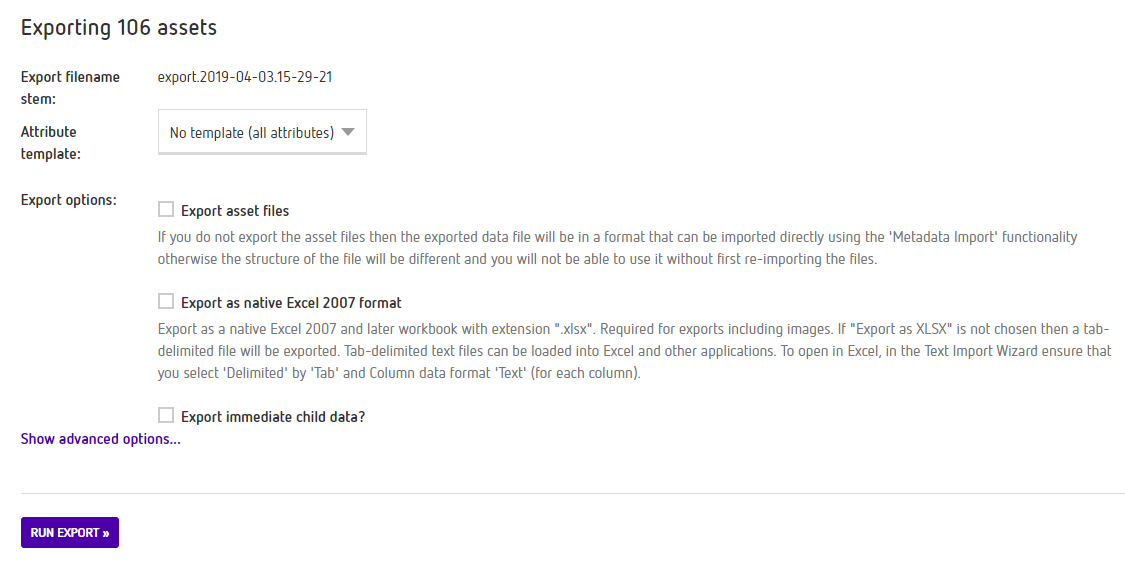The image showcases a page with a white background, densely populated with text. The most prominent text, located in the top left corner in bold, reads, "Exporting 106 Assets." Beneath this header, there is a section on the left side where bold text, slightly smaller in size, indicates "Export File Name Stem," followed by "Export.2019-04-03.15-29-21."

Progressing downwards on the left, another bold heading says, "Attribute Template," accompanying a drop-down box to the right that displays "no template, all attributes" with a pull-down arrow next to it. Further down, another bold heading reads, "Export Options," with three corresponding export choices aligned across from it. Each option has an adjacent box that remains unchecked.

The first option is "Export Asset Files," which contains an explanatory note specifying that not exporting the asset files results in an exported data file formatted for direct import using the Metadata Import functionality. It further explains that exporting asset files alters the file structure, necessitating re-importation prior to use.

The second option reads "Export As Native Excel 2007 Format," followed by the third option, "Export Immediate Child Data."

Continuing downward on the left side of the page, the text in bluish-purple says, "Show Advanced Options..." and in the lower-left corner, there is a bluish-purple button labeled "Run Export."